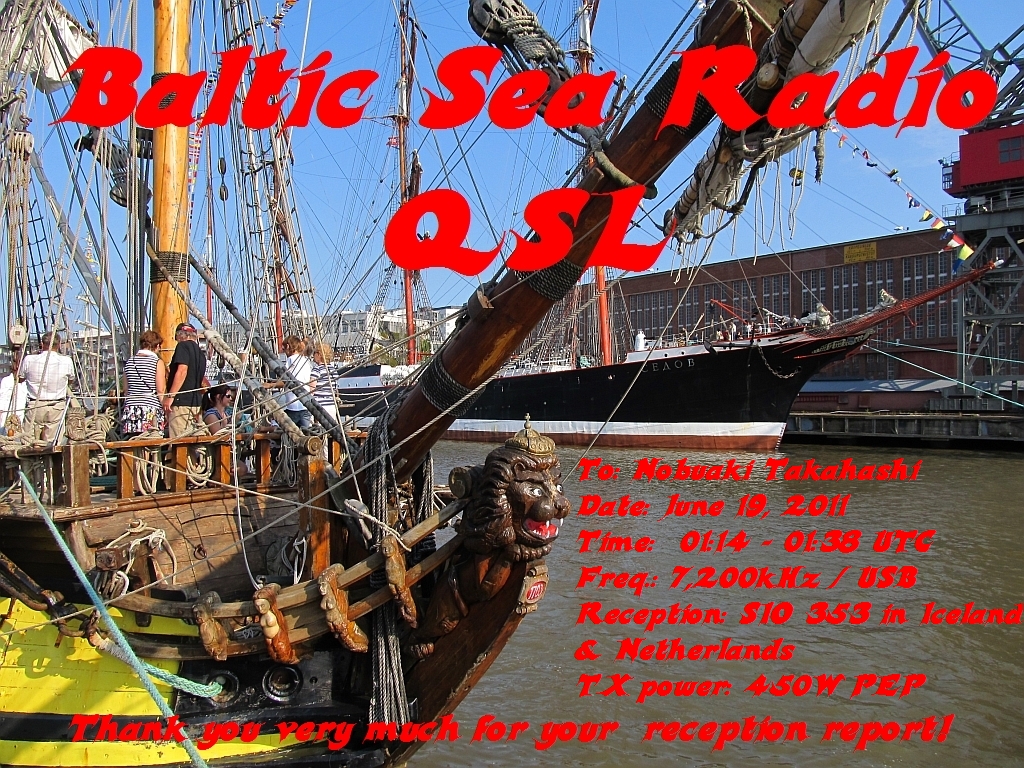The thank you card for a reception report features an outdoor photograph capturing a historic scene at a marina. The background showcases a dock lined with old-fashioned boats, prominently featuring a sailboat with multiple rigging and a carved lion on its bow. Imposed over the image is bold red text, reading: "Baltic Sea Radio QSL2, Nobuaki Takahashi, June 19, 2011, 01.14 to 01.38 UTC, Frequency 7200 kHz/USB, Reception S10353 in Iceland and Netherlands, TX Power 450 watts PEP. Thank you very much for your reception report." The text stands out against the photograph, adding a promotional flair.

On the dock alongside the sailboat, people in summer attire—shorts and short sleeve shirts—are milling about. In the background, a modern black-hulled ship with two tall masts is docked, reinforcing the maritime setting. This ship is juxtaposed against a long brick building with numerous windows, possibly a dock warehouse. The entire scene is illuminated by a bright, clear blue sky, adding vibrance to the historical and nautical ambiance of the image.